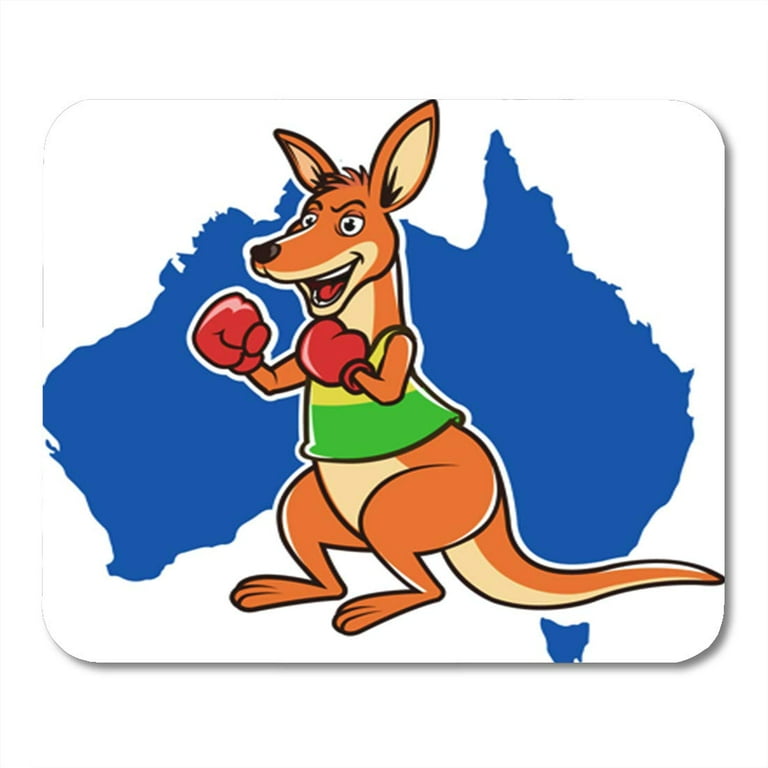This image features a cartoon illustration of a kangaroo with a cheeky, somewhat mischievous expression, suggesting it is ready for a fight. The kangaroo sports brown boxing gloves and a sleeveless tank top with green and yellow sections—green at the top and bottom. Its body is depicted in varying shades of brown, with some descriptions mentioning an orange tint, and the typical proportions of a kangaroo's legs and tail are maintained. The creature has big ears, a black nose, and a mouth open in a friendly, albeit taunting, smile. In the background, there's a solid blue silhouette of the Australian continent set against a white backdrop. The image is framed within a rectangular outline with rounded edges. This playful and vibrant design could serve excellently as a school or team mascot, bringing a spirited and lively character to any organization it represents.